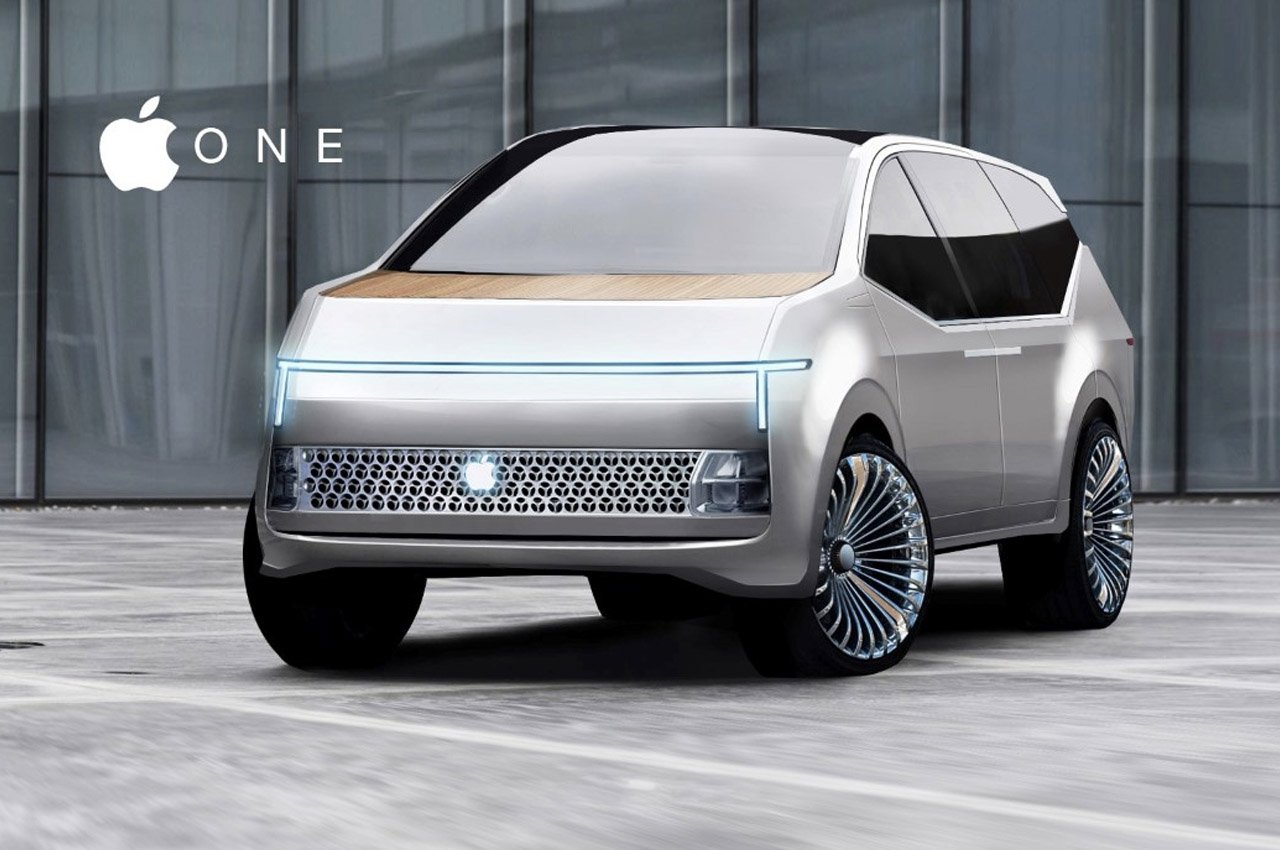The image features an Apple-branded electric vehicle concept, prominently displayed in an advertisement or product poster. In the upper left-hand corner, the iconic bitten Apple logo appears in white, accompanied by the text "Apple One," suggesting the vehicle’s name. The car itself, with a sleek and futuristic SUV design, is a striking silver or light gray, almost chrome-like shade with a hint of light gold.

The vehicle is positioned on a stark gray surface, possibly resembling a showroom floor, and it overlaps what could be parking spots, adding to the sense of its grand presence. The background features a slightly darker, mysterious material—either metal or glass—enhancing the minimalist aesthetic.

Key details include black-tinted windows, offering no visibility into the interior, and a grille adorned with an illuminated Apple logo amidst silver spindles. The hood sports a subtle wood panel design, adding a unique touch to its modern appearance. The wheels are particularly eye-catching, each with multiple bright, silver spokes that contribute to the vehicle’s distinctive and memorable look.